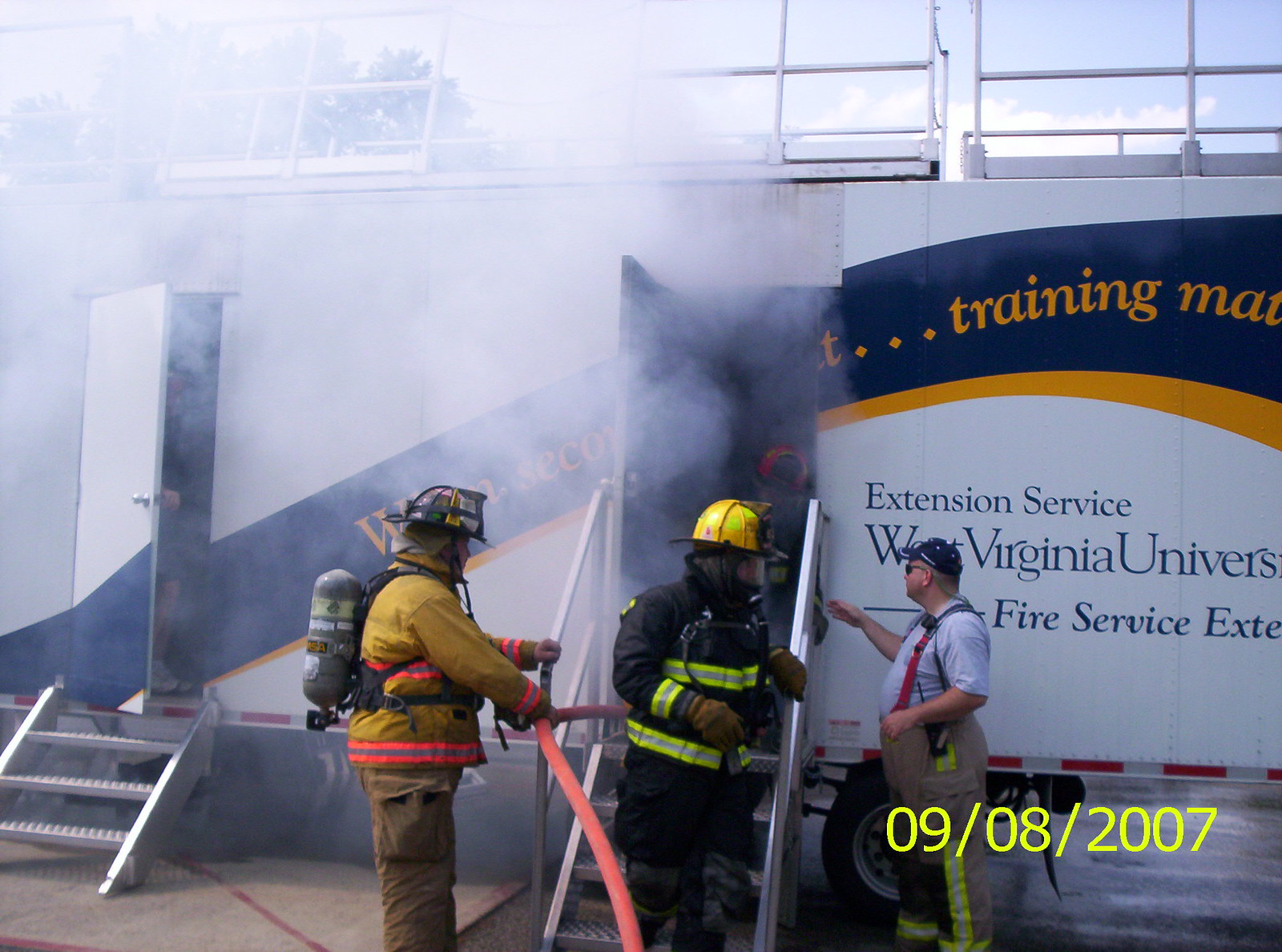This color photograph, taken on a bright day on September 8, 2007, showcases a detailed scene of an intensive firefighting training session at the West Virginia University Fire Service Extension. The image, in landscape orientation, captures a white, repurposed shipping container used for simulating fire scenarios. Two metal steps lead up to the double doors of the container, both of which are open with thick, billowing smoke pouring out, emblematic of a controlled fire exercise. 

At the forefront of the scene are three individuals: a central figure wearing a yellow hard hat and a black overcoat with green striping, identified as the instructor, flanked by two firefighters. On the left stands a firefighter dressed in a gold jacket, helmet, and carrying a red fire hose, while another man on the right sports a blue short-sleeve shirt with red suspenders. They are all positioned in front of the container, which features clear white graphics and a dark blue swash with gold lettering that includes the words “Extension Service” and “West Virginia University Fire Service Extension.” 

The setting appears to be a parking lot or a training ground with metal scaffolding visible above the container. The realism of the photograph emphasizes the structured and methodical approach taken in firefighter training, capturing a critical moment in the instruction of emergency responders.